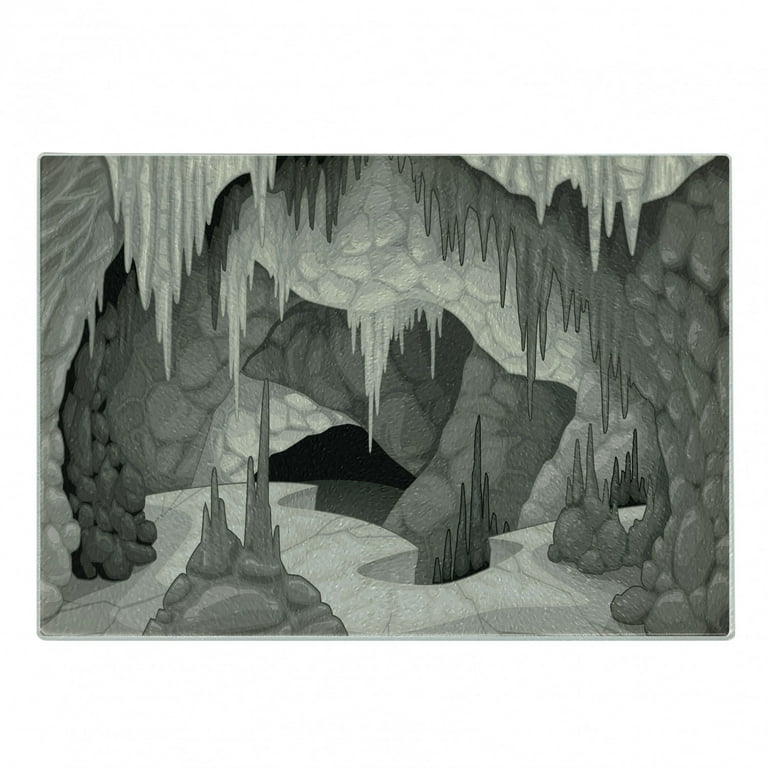This image is a detailed black-and-white illustration, likely intended for an animation. It features a cave interior with various intricate formations. The drawing is rectangular, about five inches wide and three inches high, encased in a light gray beveled border. The cave's ceiling and floor are adorned with numerous stalactites and stalagmites, suggesting a dripping, almost melting appearance. 

The upper area of the cave has icy-looking stalactites hanging down, while the right side of the cave displays stone formations that appear to merge or stack together to form a wall. These formations project leftward, casting different gray and white shades. The cave floor in the immediate foreground is flat with ice-like texture and visible cracks, transitioning into dark gray stones with stalagmites rising upward.

Toward the center, a significant drop-off or cliff plunges into a deeper, black abyss, giving an impression of either a descending passageway or an opening into a night sky. The overall composition creates an arch-like structure formed by the overhead formations, leading the viewer's eye to a vanishing point in the darker, lower-left section of the image. The grayscale shading enhances the depth and mystique of the cavern.